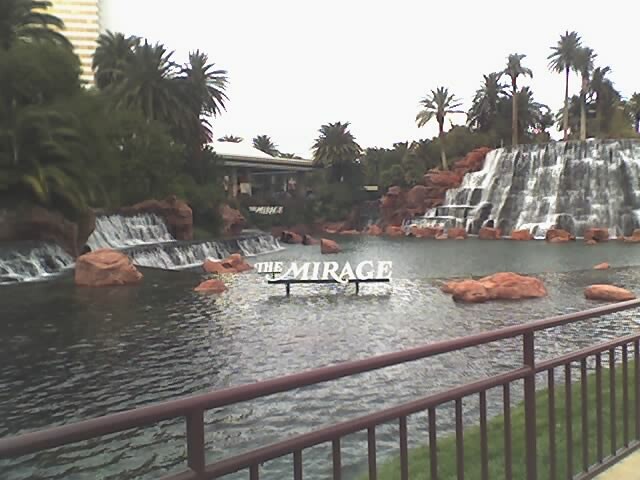The photo captures the exterior of the old Mirage Casino, showcasing a scenic, man-made lagoon adorned with waterfalls and large boulders. Prominently featured in the center of the water is a white sign that reads "The Mirage," positioned on a platform or bench. Surrounding the lagoon are lush groups of palm trees and tropical plants, enhancing the resort's aesthetic. Visible in the distance, to the top left, is a towering skyrise hotel building. Nearby, a fence acts as a barricade, adjoining a pedestrian walkway. Overcast skies cast a gray hue over the scene, adding a subdued atmosphere to the otherwise vibrant resort area.